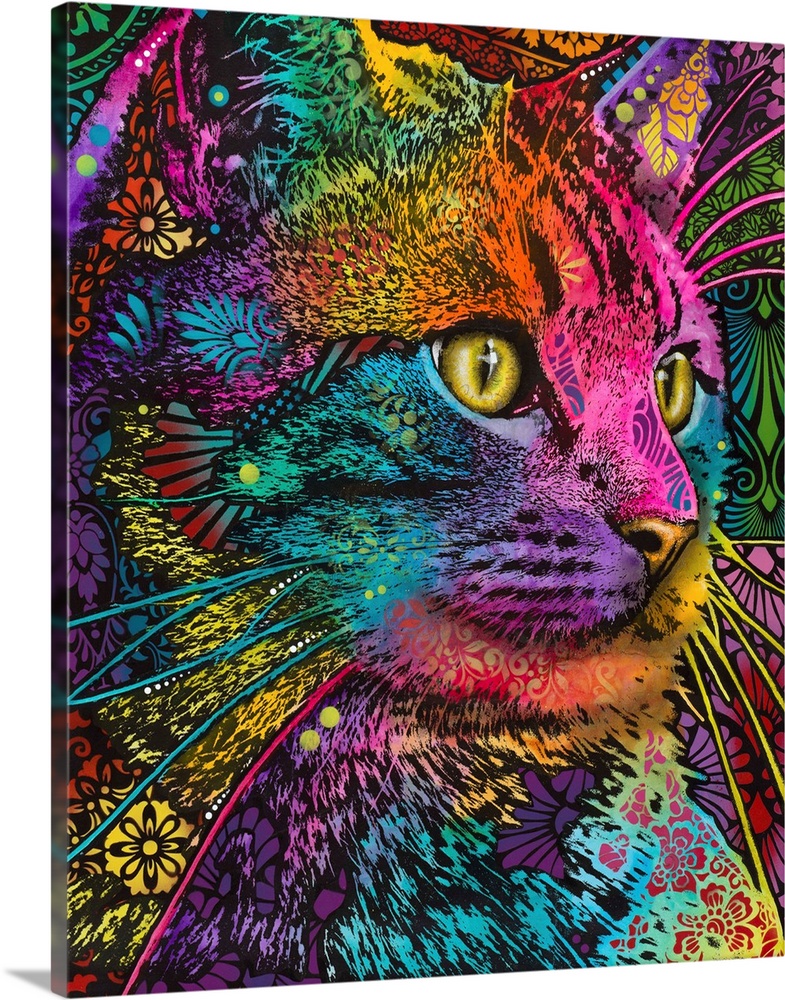The image is a vibrant, psychedelic art print of a cat, designed as a digital canvas wrap with a 3D effect. The cat, positioned in a three-quarter turn facing to the right, features an array of neon colors including purples, turquoises, pinks, oranges, yellows, and hot pinks, creating a rainbow-like appearance. Its erect ears, bright yellow eyes, and textured whiskers add to the intricate detail. The fur is composed of diverse brush strokes and abstract shapes, adding to its psychedelic nature. Floral patterns, lace-like textures, and symbols such as butterflies and geometric designs adorn the background and the cat itself, contributing to the image's overall vibrant and engaging quality. The background, filled with similar colorful and textured elements, enhances the dynamic aesthetic of the artwork.